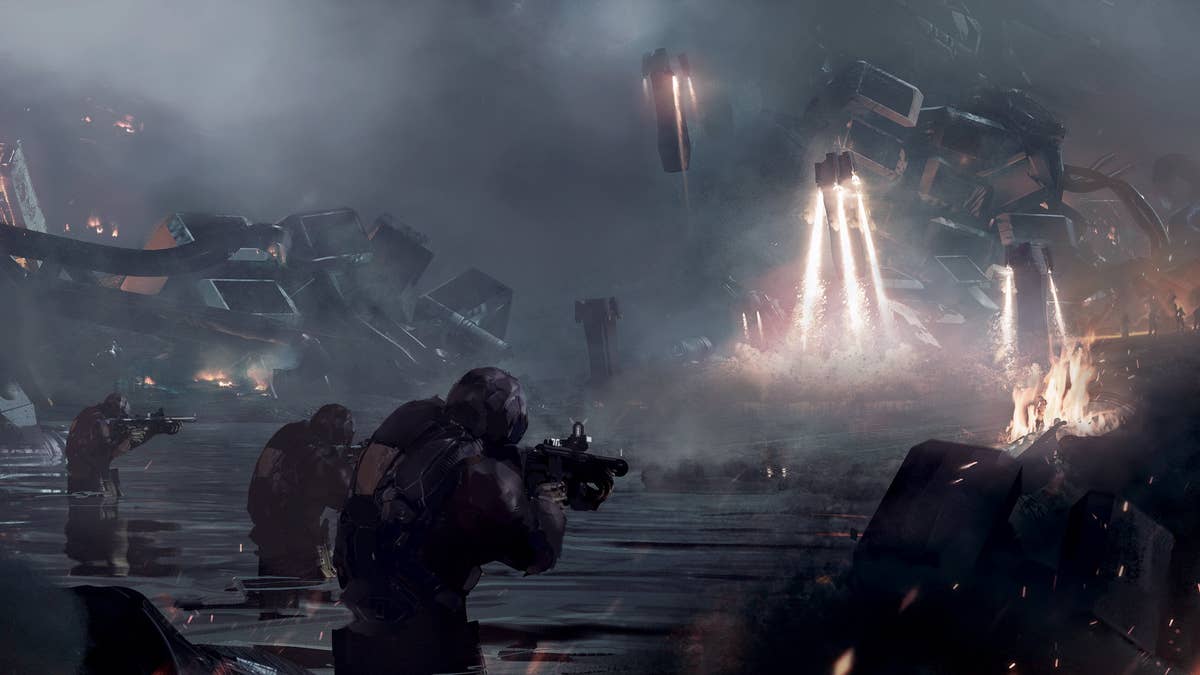The image depicts a highly detailed, chaotic science fiction scene reminiscent of a futuristic movie or video game like Fortnite or Call of Duty. Set in a dark, nighttime environment with an overwhelming sense of destruction, three heavily armored soldiers in the foreground stand knee-deep in water. They are dressed in heavy coats and camouflage, complete with helmets, and are aiming their high-powered rifles at an enigmatic, monstrous machine that resembles a dinosaur-rocket hybrid. This mechanical creature has a face, squared arms, and is emitting three flames from each arm, as if outfitted with flamethrowers.

The background is filled with rubble, illuminated sporadically by lights that cast eerie shadows across the scene. To the right, a vast expanse of darkness conceals several indistinct machines, while the left reveals more machinery, some parts broken or destroyed, lying carelessly in a heap. The atmosphere is thick with smoke and haze, adding to the sense of urgency and conflict. Additional soldiers can be seen further in the distance, also moving towards the mechanical adversary, contributing to an overall impression of a large-scale battle unfolding in a dystopian setting.